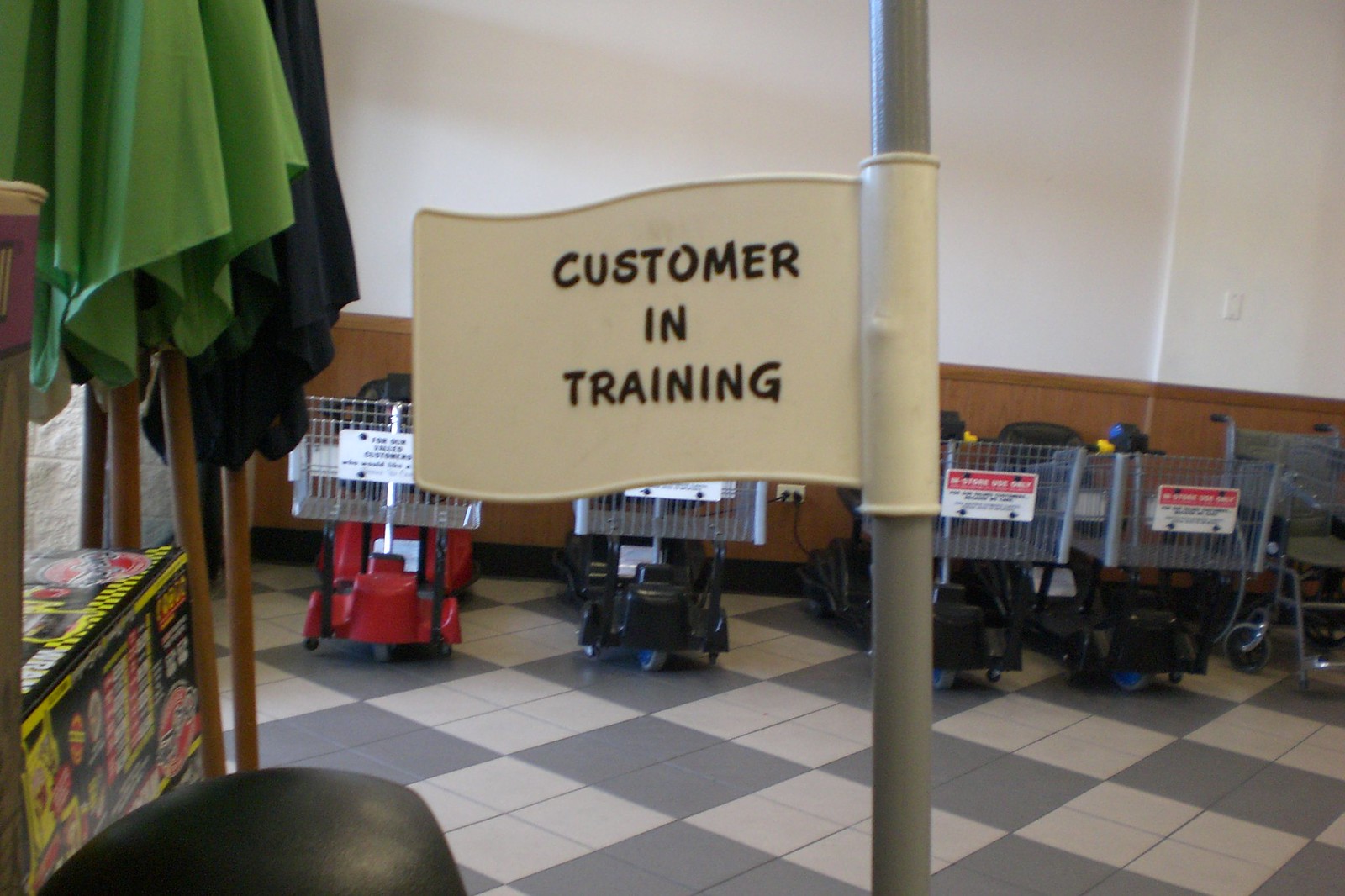This vibrant color photograph captures a section of a store or supermarket. The scene features a neatly arranged line of motorized shopping carts positioned against a two-tone wall; the lower portion of the wall is brown while the upper portion is white. Dominating the right center of the image, a vertical pole is prominently visible. Attached to this pole is a plastic flag emblazoned with the text "Customer in Training" in black lettering. To the left side of the image, several black and green summer umbrellas with brown frames lean casually against the wall. Below these umbrellas, there is a boxed item, likely a toolset. Sunlight streams in from the left side of the image, casting a natural light through a door or window behind the umbrellas, enhancing the warm and inviting ambiance of the scene.